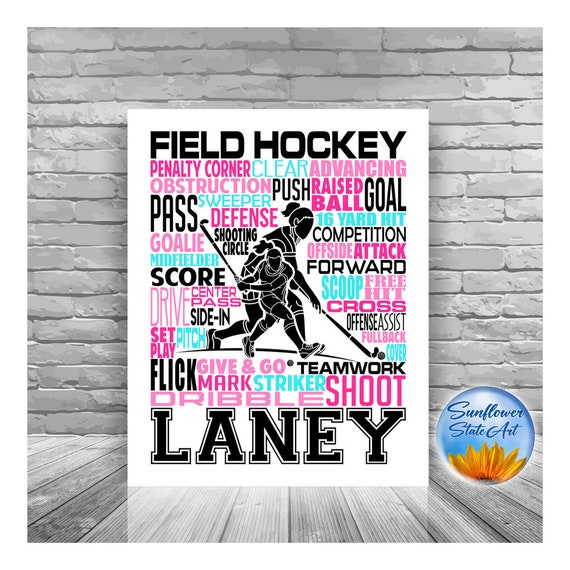This image is a detailed color photograph of a custom-made field hockey-themed graphic poster. It is positioned against a backdrop of a white brick wall and rests on a black and white hardwood floor. The poster itself features a vibrant array of field hockey terminologies and phrases in pink and light blue, such as penalty corner, clear, advancing, obstruction, push, raised ball, goal, pass, sweeper, defense, 16-yard hit, goalie, shooting circle, competition, offside, attack, forward, scoop, free hit, cross, offense, assist, fullback, score, drive, center pass, side-in, set play, pitch, flick, give, give and go, teamwork, mark, striker, shoot, and dribble. At the top of the poster, the words "Field Hockey" are prominently displayed in black, while at the bottom, the name "Laney" is also written in black. The background of the poster is white, adding a clean contrast to the colorful text. On the bottom right corner of the poster, there is a distinctive blue 3D circle featuring an emblem and the label "Sunflower State Art," with a sunflower design within the circle. The overall aesthetic of the image is enhanced by the reflective quality of the hardwood floor beneath the poster.